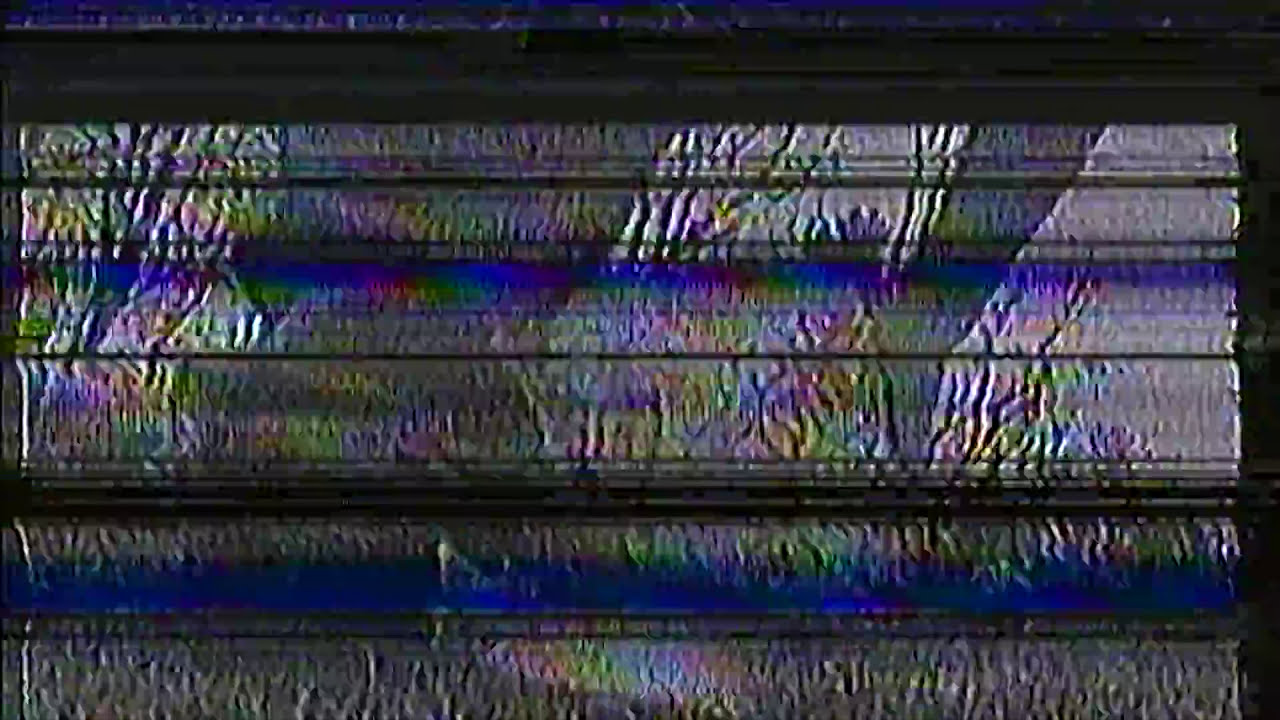Viewed through the distorted lens of horizontal blinds, this photograph resembles an abstract painting. The image captures a scene marked by the gray and black hues of a metallic or reflective surface, with streaks of rainbow colors—like blue, pink, yellow, and green—evoking the iridescent sheen of an oil spill. These colors, combined with the textured and slightly transparent appearance of the blinds, create a surreal, almost holographic effect. Amidst this distortion, two trees can be discerned outside the window: one with a thick trunk on the left and a thinner one, adorned with more colorful growth, on the right. Black border lines frame the image, adding to its static, pixelated quality, reminiscent of an old, low-quality television screen. The overall composition, with its mixture of shadows and light-reflective elements, transforms a simple outdoor view into an enigmatic visual abstraction.